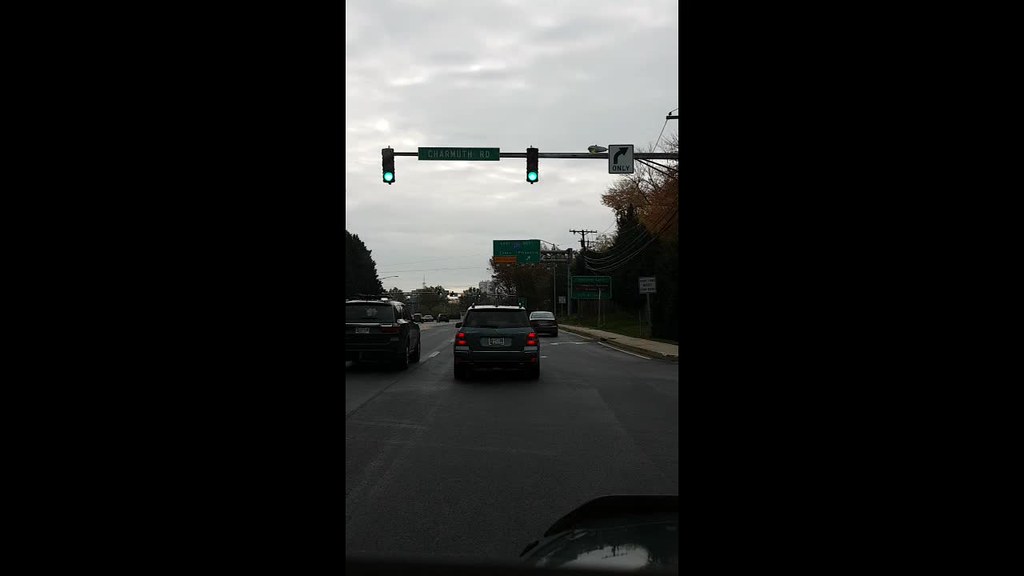The image captures a narrow view through the front window of a car, framed by approximately six inches of black space on either side, possibly indicating the use of a dashcam with a limited field of view. Central to the scene is a traffic light that is prominently glowing green, with a "Right Turn Only" sign directly below it, indicating lane directions.

To the right side of the image, a green street sign with white lettering can be seen, which appears to read "Charmuth Road." Flanking this area are several trees and directional signage. No billboards are visible, but there is an upcoming green sign providing lane instructions.

On the left, only a sparse line of trees is visible. The road ahead is occupied by multiple vehicles: one car is in the right-turn lane, while two others are in separate lanes heading straight. A station wagon is leading the central lane, with a hatchback positioned to its right.

The sky appears ominous, heavy with dark clouds that hint at impending rain, setting a somewhat gloomy atmosphere for the scene. Overall, the road stretches ahead under a brooding sky with a few scattered vehicles navigating their respective lanes.